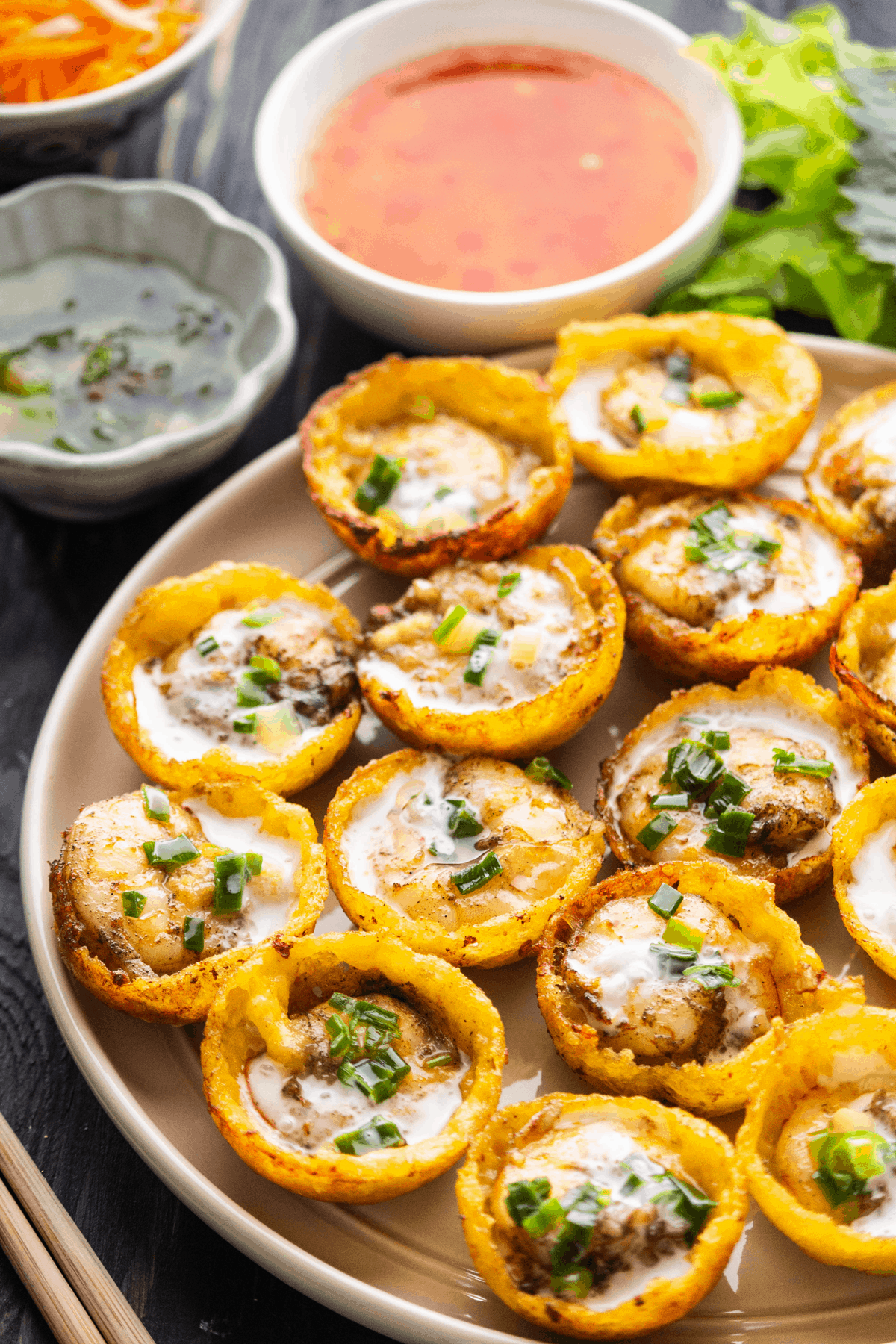A rectangular photograph showcases an artful display of food, capturing a variety of appetizing elements arranged neatly on a restaurant table. In the foreground, a wide, round brown plate holds an array of 18 individual hors d'oeuvres, each resembling fluted cups made of cornmeal or pastry. These circular cups are filled with a tantalizing creamy mixture, possibly involving scallops or mushrooms, and are generously topped with melted cheese and finely minced chives. Behind this platter, in the upper left corner, are three distinct bowls that complement the main dish. The topmost bowl contains thin slices of orange material, likely carrots or cheese. Below it, a gray bowl is filled with a green, murky liquid, which could be a vinaigrette or some sort of tapenade. The third and largest bowl, white in color with lettuce adorning its rim, holds an orange-toned sauce that could be chili oil or another flavorful dipping sauce. Decorative greens are also scattered about, enhancing the overall presentation.